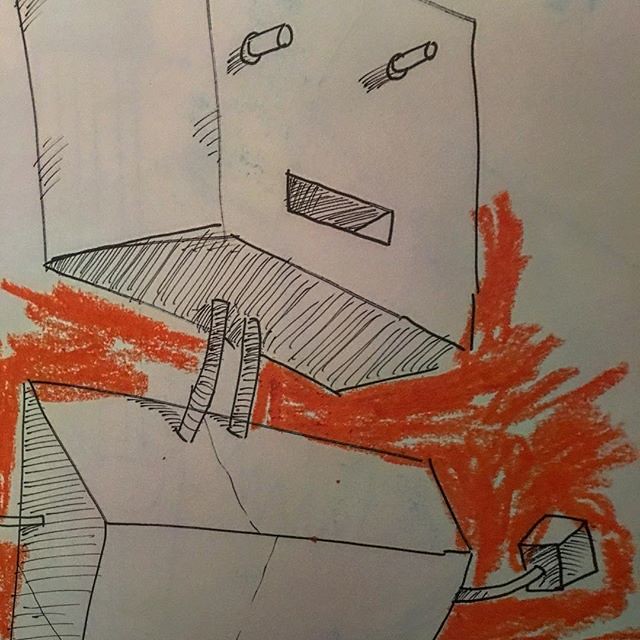This hand-drawn illustration features a robot meticulously sketched with markers on white paper. The robot's square head includes a rectangular, shaded-in mouth and cylinder-like bolts serving as eyes. Its head is connected to the rectangular body by two thin wires. An orange hue accentuates the lower part of the robot’s neck and extends onto its body. One of the robot's hands is depicted with a square block-like structure, which has also been shaded for depth and dimension.